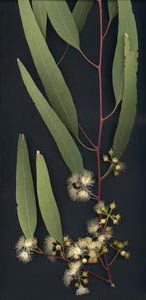This detailed image depicts a slender, reddish-brown vine or stem set against a completely black background. Extending from this stem are about ten long, narrow leaves that vary slightly in shades of light and dark green. These leaves are arranged along the vine, almost appearing to branch out from it. At the very base of the stem is a cluster of fluffy, seed-like protrusions that are white and grayish cream in color. Some of these blooms are fully opened, resembling thistledown or dandelion fluff, while others remain as small buds. The contrast between the delicate texture of the blooms and the elongated, sleek leaves alongside the dark background creates a visually striking botanical study.